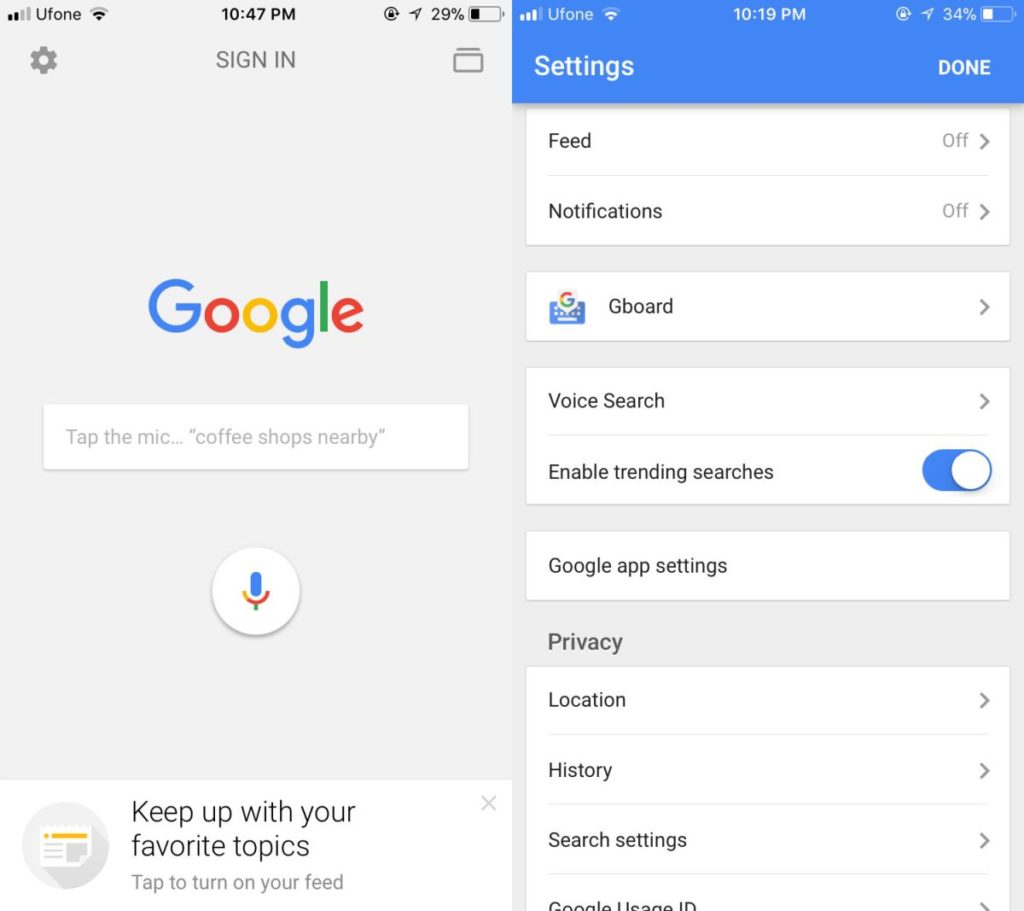This image showcases two cell phone screens side by side, displaying different interfaces.

On the left, the screen presents a user interface with a gray background. In the top-left corner, "U Phone" is displayed, while the center shows the time "10:47 PM." Beneath the time, there is a gear icon and the words "Sign in." Further down the screen, "Google" is prominently displayed above a text box with the phrase "Tap the mic" and the example query "coffee shops nearby" in quotes. Below this text box, there is a circular icon featuring a microphone. Lower down, an image of a newspaper is accompanied by the text "Keep up with your favorite topics. Tap to turn on your feed."

The screen on the right is displaying the settings page. At the top, it reads "Settings" followed by "Feed," which is toggled to "Off." "Notifications" is listed next, also set to "Off." Below these, a keyboard icon with the Google logo is labeled "Gboard." The subsequent option is "Voice Search," followed by "Enable trending searches," which is activated. Under this, "Google app settings" is listed. The following category, labeled "Privacy," includes several options: "Location," "History," "Search settings," and a partially visible entry labeled "Google usage ID."